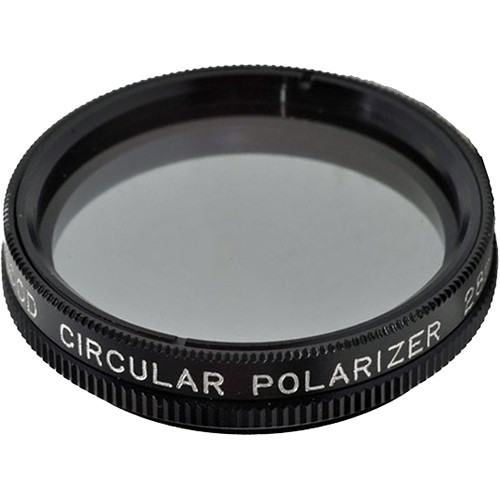Displayed against a completely white background, this image showcases a camera lens with a robust black plastic or possibly metal circumference that features a distinctive ribbed texture along both the top and bottom edges. The central glass part of the lens is a light gray color, exhibiting a reflective surface that mirrors the outer rim. Prominently engraved in white, capitalized letters on the rim is the text "CIRCULAR POLARIZER 28," though additional text exists on either side, it is not fully visible in the image.